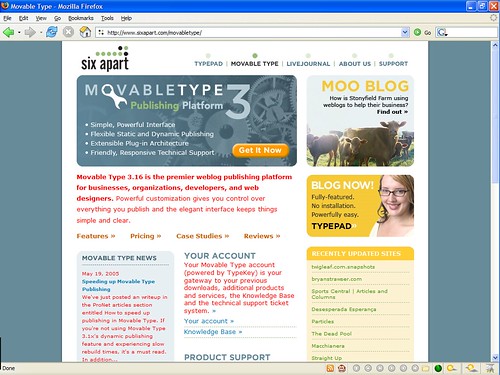This is an image of the Six Apart website displayed on the Mozilla Firefox browser. At the top, there is a blue rectangular navigation bar with "Mozilla Firefox" written next to "Movable Type." Below this, the menu options are listed as follows: File, Edit, View, Go, Bookmarks, Tools, and Help, along with various computer icons and a URL address bar.

In the main section of the webpage, "Six Apart" is prominently displayed with green and black circular logos above it. Adjacent to this are links labeled TypePad, Movable Type, LiveJournal, About Us, and Support.

A blue banner beneath this section reads "Movable Type 3 Publishing Platform," with the letter "O" stylized as a wrench. Accompanying this banner is a "Get It Now" button.

The central part of the page provides detailed information about the website, outlining sections on Features, Pricing, Case Studies, and Reviews. To the right of this information are two distinct images. The first is a square image featuring several cows with the title "MooBlog." The second is a rectangular, yellow-hued image that advertises "Blog Now, Fully Featured, No Installation, Powerfully Easy, TypePad," depicting a smiling woman with glasses and a white shirt.

The remainder of the page is filled with additional information about the website and its offerings.